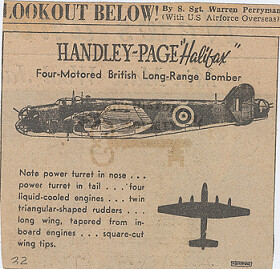The image titled "Look Out Below" by Staff Sergeant Warren Perryman from the U.S. Air Force Overseas features a detailed depiction of the Handley Page Halifax, a British four-motored long-range bomber from World War II. The centerpiece of the image is the meticulously sketched aircraft, prominently placed in the center. The plane is horizontally oriented, with its front facing the left of the image. The aircraft's long and streamlined body is highlighted, along with key features such as a nose and tail power turret, four liquid-cooled engines, twin triangular-shaped rudders, long tapered wings extending from the inboard engines, and square-cut wingtips. The colors are primarily tan, black, and gray, giving the image a vintage, sepia-toned appearance as though it were part of an old, slightly yellowed newspaper or magazine article. The setting suggests the poster is an informational or promotional piece for the military aircraft, emphasizing its design and technical specifications. In addition to the primary drawing, another smaller image of the airplane, shown flying upward to the right, appears to complement the overall layout.